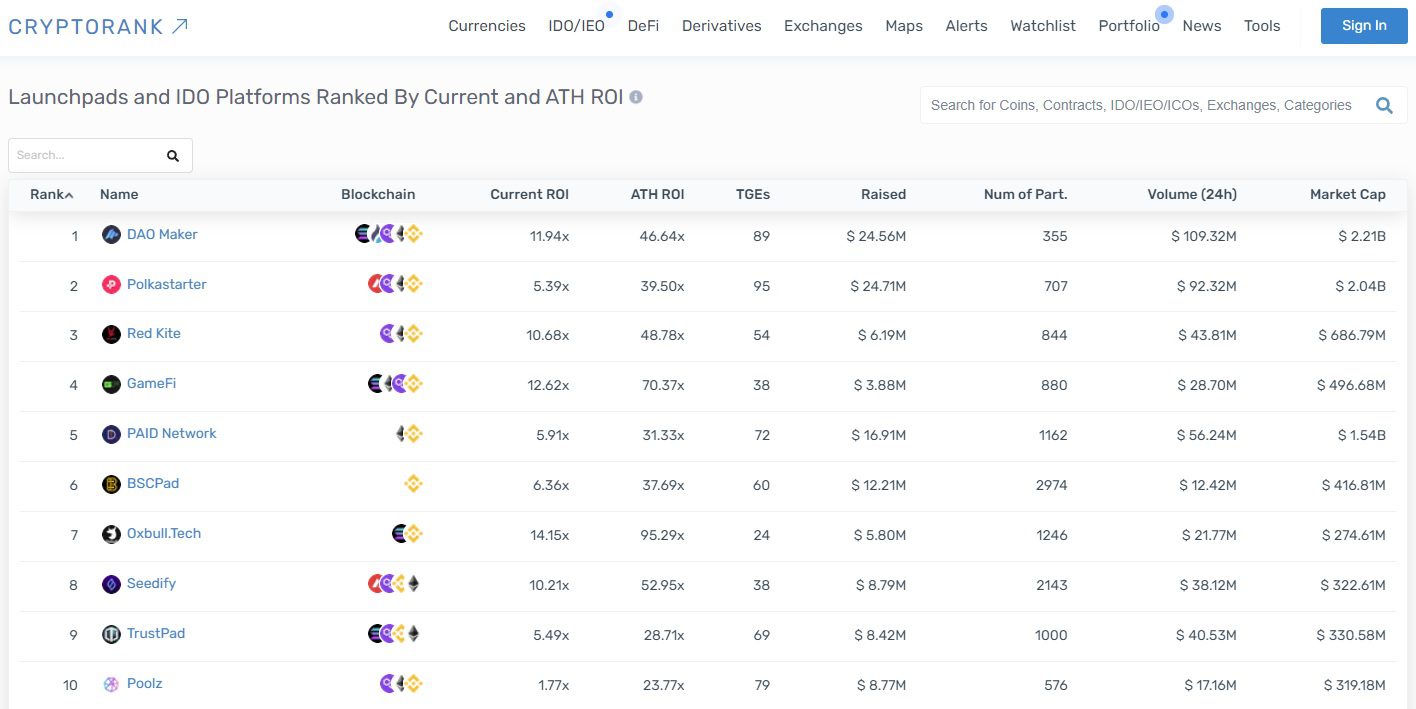Here is the cleaned-up and detailed caption:

---

In this screenshot from the Cryptobank website, the title "Cryptobank" is prominently displayed. To the right, a blue diagonal arrow pointing upwards leads to various navigation links including Currencies, IDO, IEO, DeFi, Derivatives, Exchanges, Maps, Alerts, Watchlist, Portfolio (indicated by a blue dot suggesting activity), News, Tools, and Sign In.

Immediately below, a section header reads "Launchpads and IDO Platforms, Ranked by Current and ATH ROI." This section features a searchable interface allowing users to filter for Coins, Contacts, IDO, Coms, Exchanges, and Categories.

The list is organized into columns labeled:
- Rank
- Name
- Blockchain
- Current ROI
- ATH ROI
- TGEs
- Raised
- Number of Participants
- Volume (24-hour)
- Market Cap

The rankings displayed are from 1 through 10, presenting detailed information about each launchpad and IDO platform, including their performance metrics and other key data.